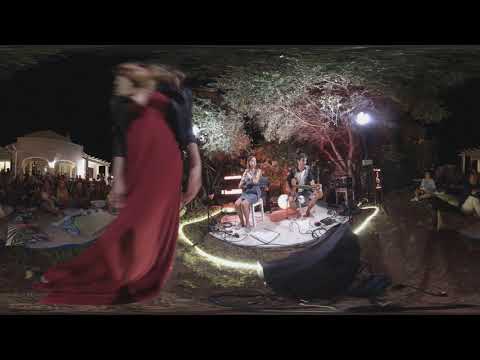The image depicts a nighttime outdoor musical performance set in a garden or front yard of a white building visible on the left. The performance space is slightly elevated, featuring white stone facing and dark tiles, and it is illuminated by overhead lights creating a bright, focused area amidst the darkness. Central to the image is a woman sitting on a white chair, holding a microphone, dressed in a blue dress. Beside her, a man with short black hair plays a brown guitar. Both are positioned on a small stage or white blanket with a ring of ground lights around them, creating a halo effect. 

To the left foreground stands a woman, possibly wearing a long red dress with black accents around the shoulders, her figure slightly blurred, and her head turned. This detail gives the image an almost surreal quality. Low to the ground on the left, two people are seated, watching the performance attentively. In the background, various trees, possibly with white-tinted leaves due to the artificial lighting, create a natural backdrop. Further right, a dirt path can be seen leading into the distance, with more observers and hints of another building partially visible. The thick black borders at the top and bottom frame the entire scene, adding to the sense of depth in the fisheye-lensed image.